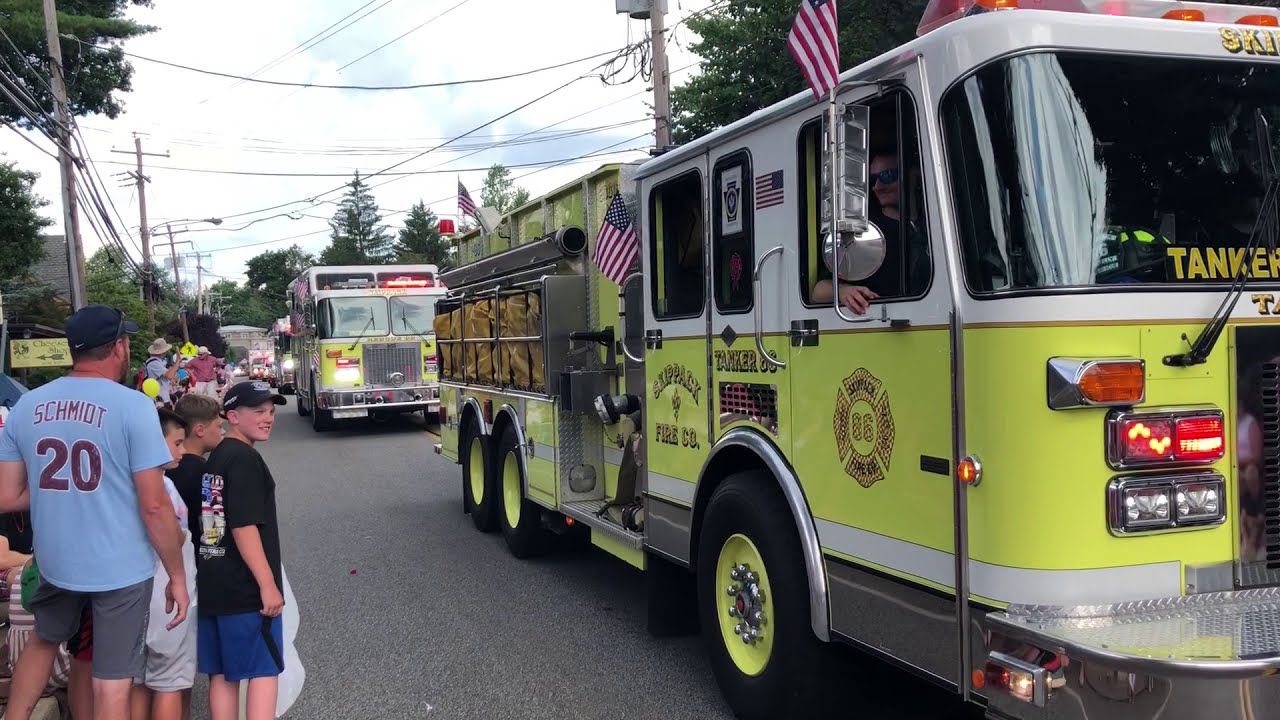The photograph captures a vibrant parade featuring a procession of distinct yellow fire trucks adorned with American flags. The leading fire truck, labeled "Tanker 86" from the Skipback Fire Company, stands out with its bright yellow and white coloration, red headlights, and yellow hubcaps. This truck is navigating a city street, where its presence is celebrated by a cheerful crowd lining the left side of the road, set against a backdrop of telephone poles and trees. Among the spectators, a man named Schmidt, identified by the number 20 on his light blue shirt and wearing gray pants and a blue baseball hat, stands with three young boys, all intently watching the parade. One boy is holding an object, adding to the scene's liveliness. Following closely behind the first truck is another yellow fire truck of a similar model, while more fire trucks and enthusiastic onlookers can be seen further down the parade route. The overall atmosphere is one of community joy and admiration for the display of fire service vehicles.